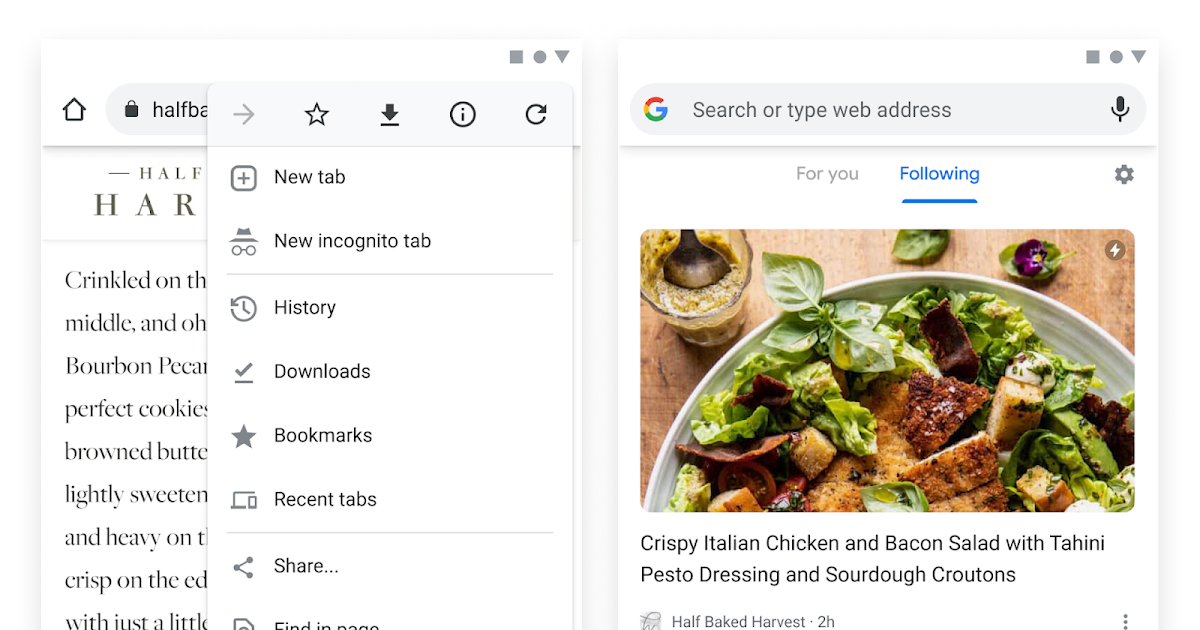The image showcases an appetizing dish artfully presented on a pristine white plate. The dish is titled "Crispy Italian Chicken and Bacon Salad with Tahini Pesto Dressing and Sardine Croutons." The succulent chicken, crisp bacon, and fresh salad components are drizzled with a rich tahini pesto dressing and garnished with crunchy sardine croutons, creating a harmonious blend of flavors and textures. On the left side of the image, the detailed recipe for this gourmet creation is visible, offering step-by-step instructions for recreating the dish at home.